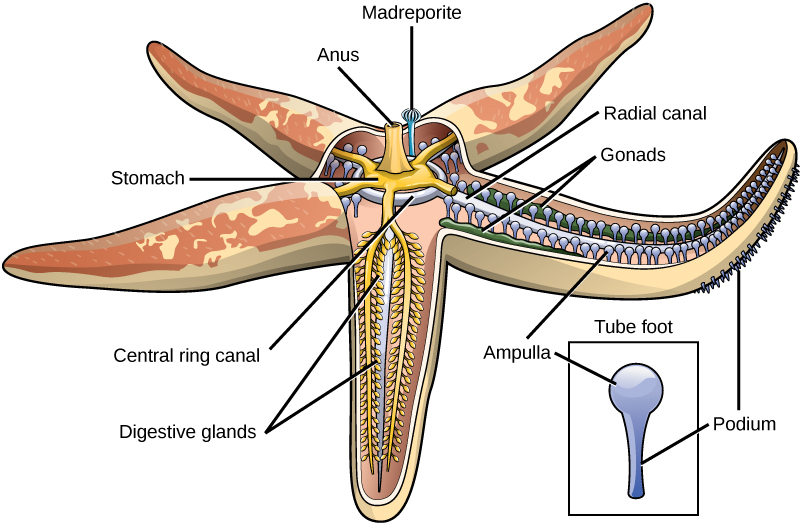This detailed illustration of a starfish, appearing digitally rendered with cell shading, offers a comprehensive view of its external and internal anatomy. The starfish is depicted in yellow with reddish and brown patches, with three of its arms shown intact, while two are cut open to reveal intricate internal structures. The labels meticulously identify various anatomical features: at the central point, we observe the madreporite, stomach, and anus. Radiating from the center are the radial canals and the digestive glands highlighted in yellow within the arms, alongside the gonads. Each leg's cross-section exhibits detailed components such as the tube feet, with the ampulla depicted as a bulbous structure and the podium as its extended part. This scientific illustration emphasizes the complexity of the starfish’s anatomy, neatly labeling features such as the central ring canal and showcasing a zoomed-in view of the tube foot system, leading to a greater appreciation of the starfish’s intricate biological makeup.